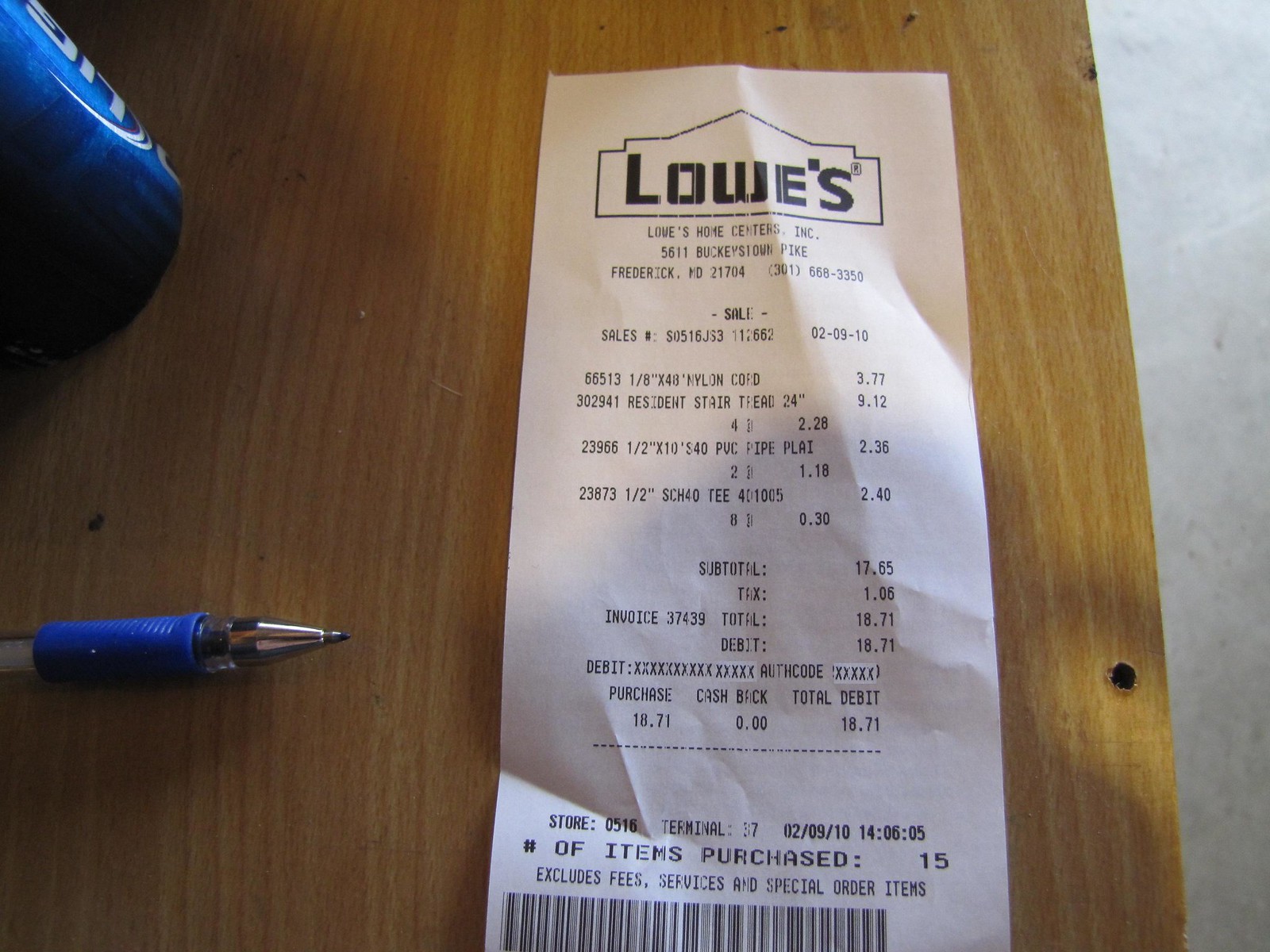A detailed photograph captures a receipt from Lowe's resting on a wooden table. To the left of the receipt, a pen with a blue barrel and a silver nib lies partially visible. Just beyond the pen, the edge of a blue bottle or can with illegible white writing can be seen. The table sits above a floor of greyish hue, noticeable on the right side of the image. The Lowe's receipt, prominently featuring the Lowe's logo in a house-shaped frame at the top, details a purchase totaling $18.17. Several lines of small, unreadable text precede a barcode and date at the bottom of the receipt. The image portrays a mundane scene with careful attention to everyday details.